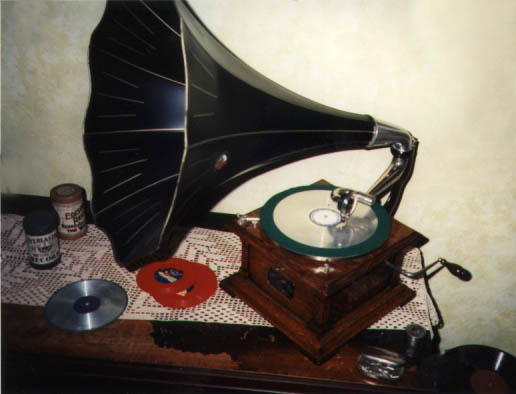This image is a personal photograph of a very old antique Victrola-style phonograph. The phonograph is a wooden box with a hand crank on the side, used to wind up a spring to play records. Attached to the wooden box is a large, silver speaker horn that extends out and then transitions into a large, black lacquered wooden horn, shaped like a cone shell, which amplifies the sound. On the phonograph, there's a shiny, silver-looking record, and surrounding it, on the table, are several other records, including a couple of red ones and a silver one. There are also a couple of jars on the table, all of which are sitting on a white lace doily. The photo itself appears to be of low quality and seems to capture the phonograph at an angle, perhaps to display it for selling or showing it off due to its rarity and historical significance.